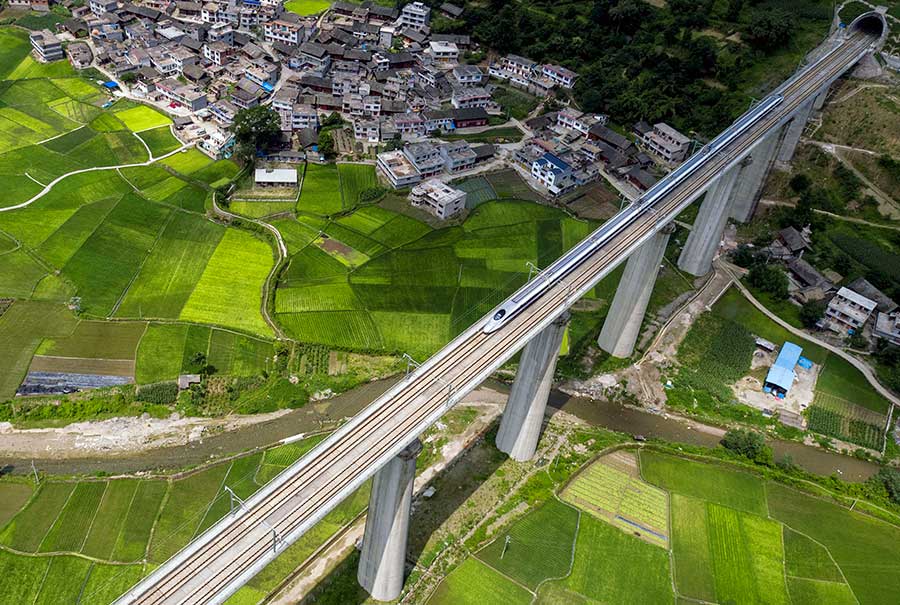This aerial photograph captures a dynamic scene featuring a sleek bullet train traversing an elevated bridge supported by massive concrete pillars. The train, running diagonally from the top right to the bottom left, cuts across the landscape. Below, vast green fields in varying shades are neatly segmented, suggesting a patchwork of farmland. In the upper left corner, a tightly clustered village with predominantly white buildings topped with black roofs stands out. The village is densely packed, with structures appearing almost stacked upon one another. A river winds its way under the bridge, completing this picturesque blend of transportation, architecture, and nature.